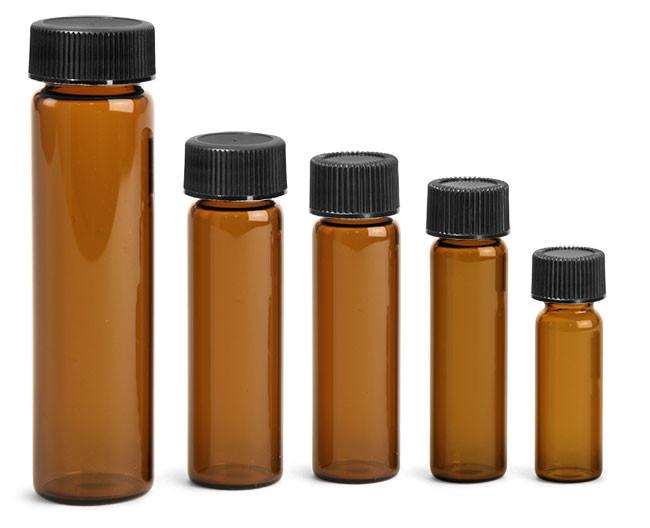The image displays five medical-style sample vials made of amber-brown, clear glass, each with a black plastic screw-on cap. Arranged in descending order of size from left to right, the largest vial on the far left stands nearly two inches tall, while the smallest on the far right measures about half an inch. Each cylindrical vial, less than half an inch in diameter, shows a reflection of light originating from the right side, alongside a faint shadow. This reflection appears larger on the vials positioned towards the left. The entire set is positioned against a stark white background, likely for a promotional photograph for a brochure or magazine, emphasizing the amber-brown and black color scheme.